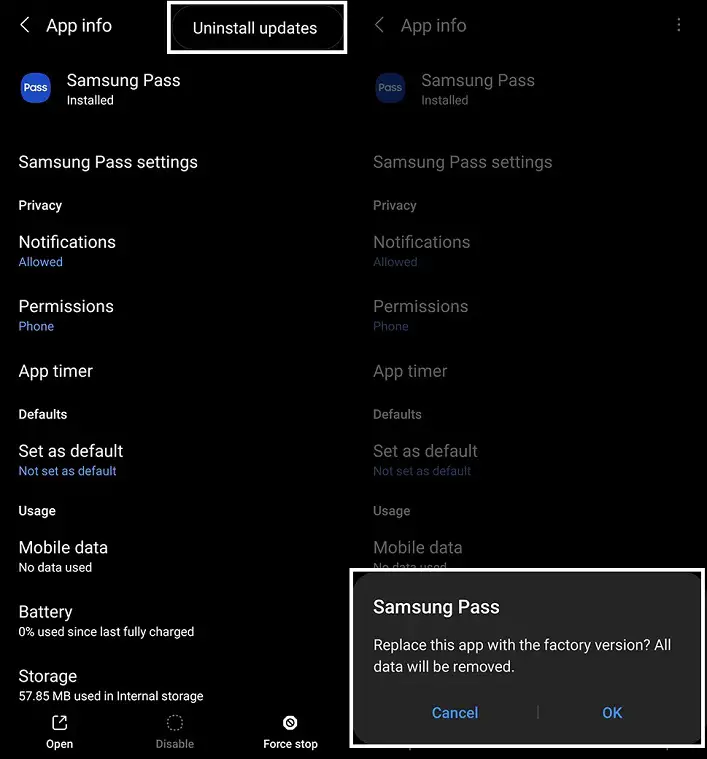This image features a composite of two screenshots displaying various settings for the Samsung Pass app. The visuals are marked by a black background with white and light blue text. 

The first screenshot, positioned on the left, showcases an "App Info" header at the upper-left corner. A white square is drawn around the "Uninstall Updates" option to emphasize it. Below this, the screen lists "Samsung Pass" as installed, followed by "Samsung Pass settings" that include adjustable categories such as Privacy, Notifications, Permissions, App Timer, Defaults, Set as Default, Usage, Mobile Data, Battery, and Storage.

The second screenshot, on the right, contains a critical pop-up in the lower-right corner, also encased within a white square. This pop-up message reads, "Samsung Pass: Replace this app with the factory version. All data will be removed." It includes options for "OK" and "Cancel" buttons. The highlighting in the first screenshot indicates that selecting the "Uninstall Updates" option leads to the confirmation pop-up shown in the second image.